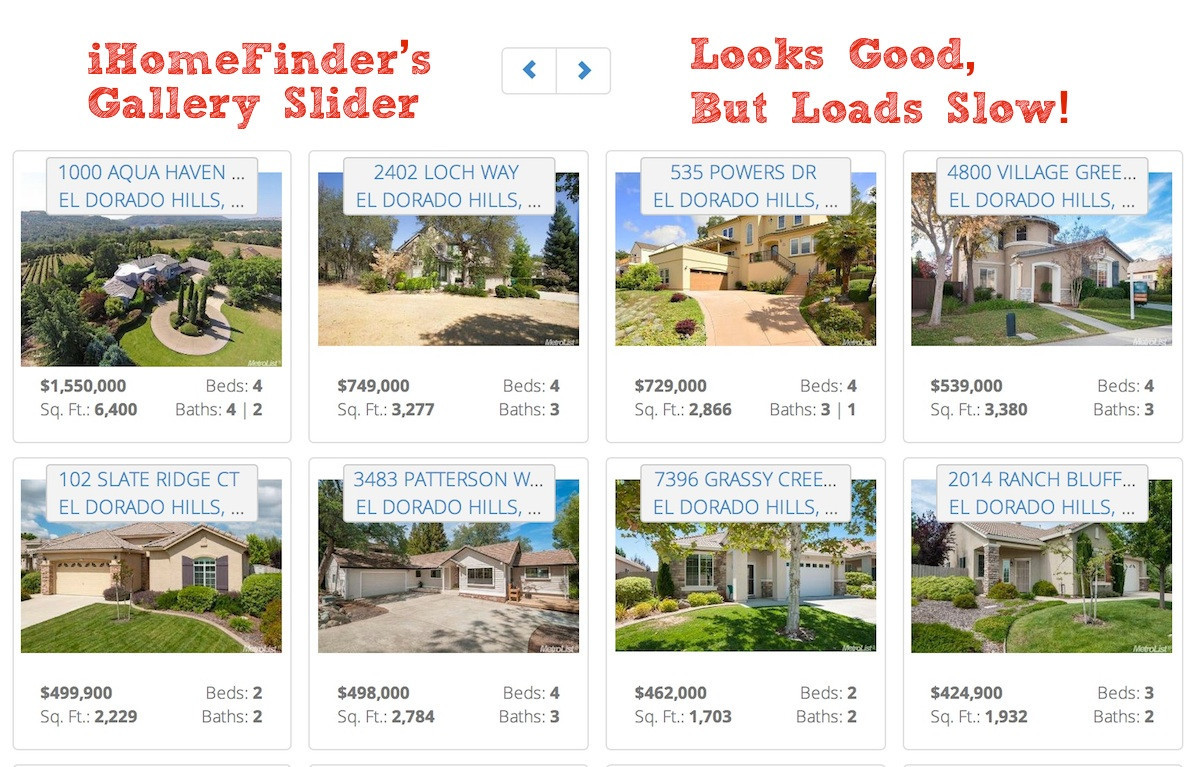A white background showcases listed properties primarily in El Dorado Hills, with notable tabs labeled as "i-Home," "Founders," "Gallery," and "Slaughter." The webpage visually appealing yet slow to load, features navigational arrows on both the left and right. Specific properties include:

1. "100 Aqua Haven, El Dorado Hills" offering four bedrooms and four bathrooms.
2. "2402 Lockway, El Dorado Hills" featuring four bedrooms and two bathrooms.
3. "535 Powers Drive, El Dorado Hills" with four bedrooms and three bathrooms.
4. "4800 Village Lane, El Dorado Hills" noted with some missing text, featuring four bedrooms and three bathrooms.
5. "102 Slate Ridge Court, El Dorado Hills" with four bedrooms and three bathrooms.
6. "3483 Patterson Way, El Dorado Hills" featuring two bedrooms and two bathrooms, partially missing text.
7. "7396 Grassy Creek, El Dorado Hills" with four bedrooms and three bathrooms, partially missing text.
8. "2014 Ranch Bluff Drive" featuring three bedrooms and two bathrooms.

All properties are majorly located in El Dorado Hills, presented with clear headings yet incomplete text on certain addresses.